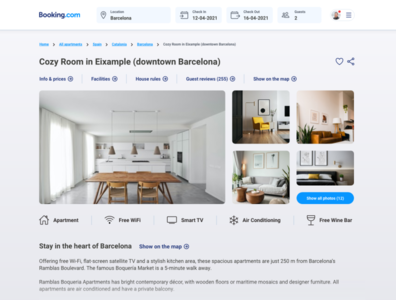**Booking.com Browsing Experience: Detailed View**

The image features a screenshot of the Booking.com website, as viewed from a desktop or laptop. At the top of the interface, the "Booking.com" logo is prominently displayed, with "Booking" in a very dark blue font against a white background, and ".com" in a lighter blue shade.

Immediately below the header, the search criteria are outlined:
- **Location:** Downtown Barcelona (Eixample)
- **Check-in Date:** 12th April 2021
- **Check-out Date:** 14th April 2021
- **Guests:** Two people

A faint profile picture with a red notification dot is visible to the right, indicating the user is logged into their profile.

The user is specifically viewing details for a "cosy room" in Eixample, Downtown Barcelona. The visual elements include a series of images showcasing the accommodation's interior:
1. **Kitchen:** Dominantly white decor except for a light wooden dining table with four matching chairs, complemented by three ceiling lights of a similar light wood color.
2. **Sitting Area:** A bright yellow armchair, likely situated in the bedroom, paired with a white couch.
3. **Bedroom:** A bed adorned with a dark black bedspread, alongside another orange-colored couch.

The overall style is very minimalistic and white-themed, providing a sleek, modern feel.

Additional amenities listed below the images include:
- Free Wi-Fi
- Smart TV
- Air conditioning
- Free wine bar

A highlighted text below these features reads, "Stay in the heart of Barcelona," with an option to "Show on the map."